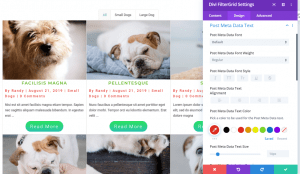This image is a blurred screenshot, likely from a blog or pet website, possibly named "Divi," "Divul," "Vowel," or a similar-sounding name, featuring fiber grid settings. The layout shows one large image at the top followed by smaller images, displaying a total of six dogs, with four dogs being mostly visible. The names of the visible dogs include Traceless, Magna, and Helen, while the others are indistinguishable. The post appears to be authored by a user named Randy, and the date is either August 21st, 2004 or 2014, though the exact year is unclear. Below the post, there's text that is too blurry to read, along with green buttons prompting readers to "read more" or access additional information. On the right side of the screenshot, there are options related to grid settings, color layout, and other website details, although the fine print cannot be made out due to the low resolution.